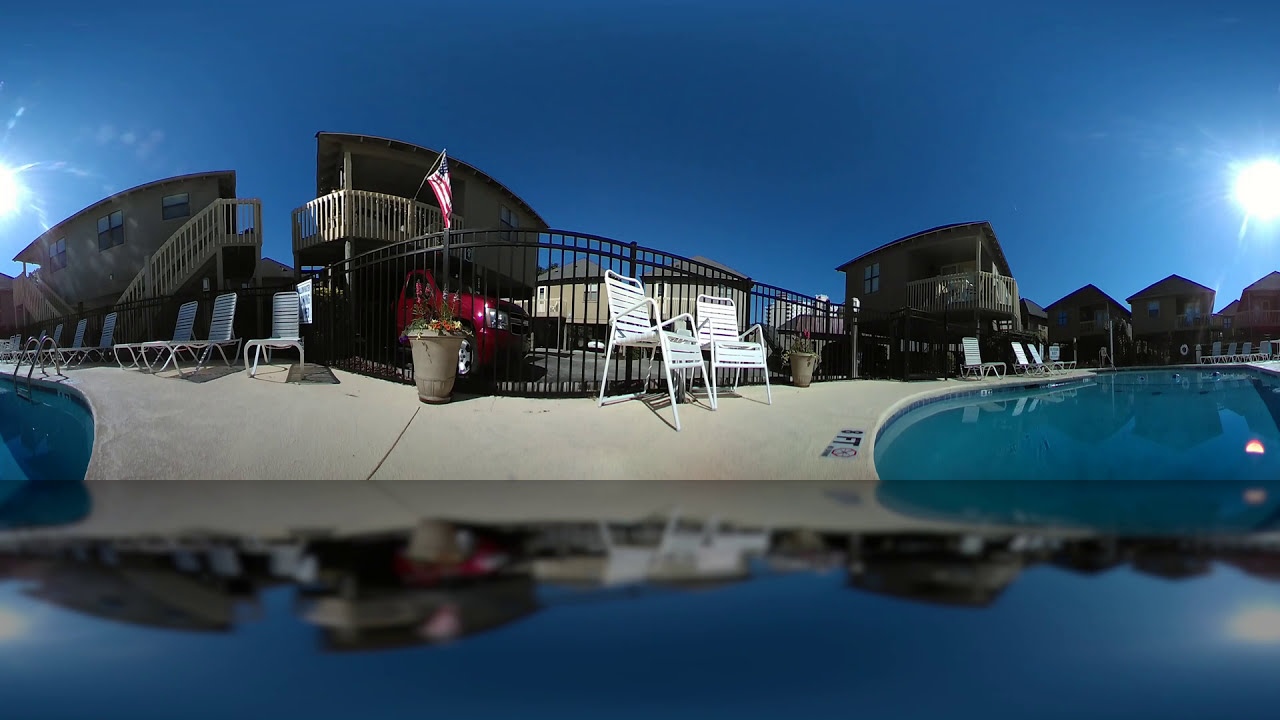The image depicts a resort-like setting captured with a fisheye lens, creating a slightly distorted view. Dominating the foreground are two swimming pools—one in the lower right and another in the left center—each bordered by concrete pathways and enclosed by metal fencing. There are 14 plastic lounge chairs with slats running horizontally across them, arranged neatly around the pools. An American flag proudly hangs from the balcony of one of several buildings, painted beige and grayish hues, which stretch across the area, reminiscent of condos or an apartment complex. These buildings feature staircases leading up to second floors and a design that includes stilts for some bungalows. A red vehicle is parked behind one of the fences, adding a splash of color to the scene. The sky above is a deep blue, marked by a bright, low-hanging sun that suggests early evening. Reflections of the scene are visible at the bottom of the image, likely cast by a reflective surface such as metal or glass, contributing to an inverted view of the surroundings.